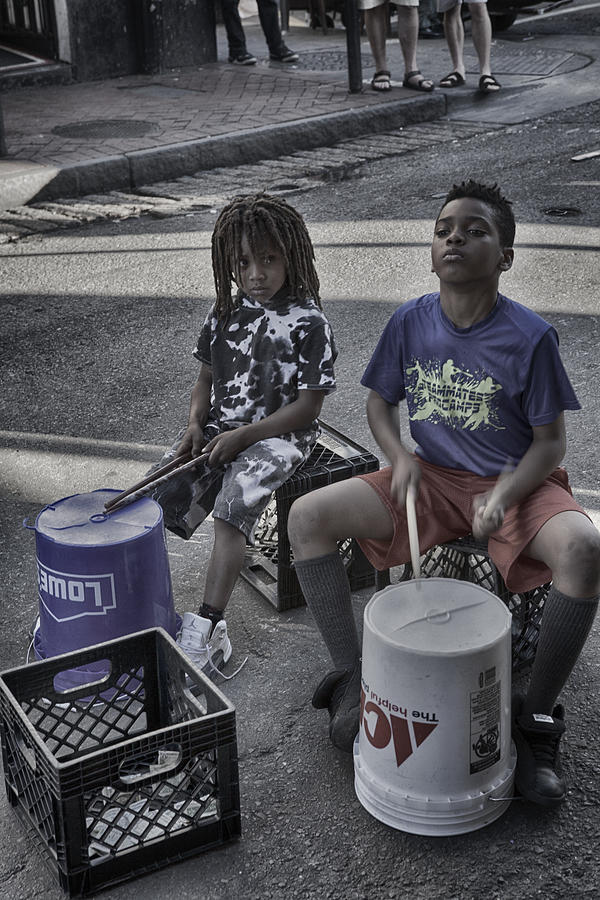In this vibrant street scene, two young boys, acting as street performers, are captured sitting on black plastic crates, energetically playing makeshift drums with a pair of drumsticks. The older boy, with light brown drumsticks, has dark complexion and curly black hair, and is dressed in a blue shirt with green accents, red shorts, gray high wool socks, and black shoes. The younger boy holds red drumsticks and has brownish-black dreadlocks, wearing a tie-dyed outfit consisting of white and black spots, complemented by white shoes and black ankle socks. They drum on two buckets, one white from Ace Hardware and the other blue from Lowe's. Scattered dollar bills are visible inside the black crates, indicating a money collection from spectators. In the background, a busy street scene unfolds with the feet of onlookers wearing sandals and shorts, standing on a red brick-paved sidewalk next to an asphalt road. The rich array of colors and the boys' lively performance lend the photo an energetic and artistic quality.